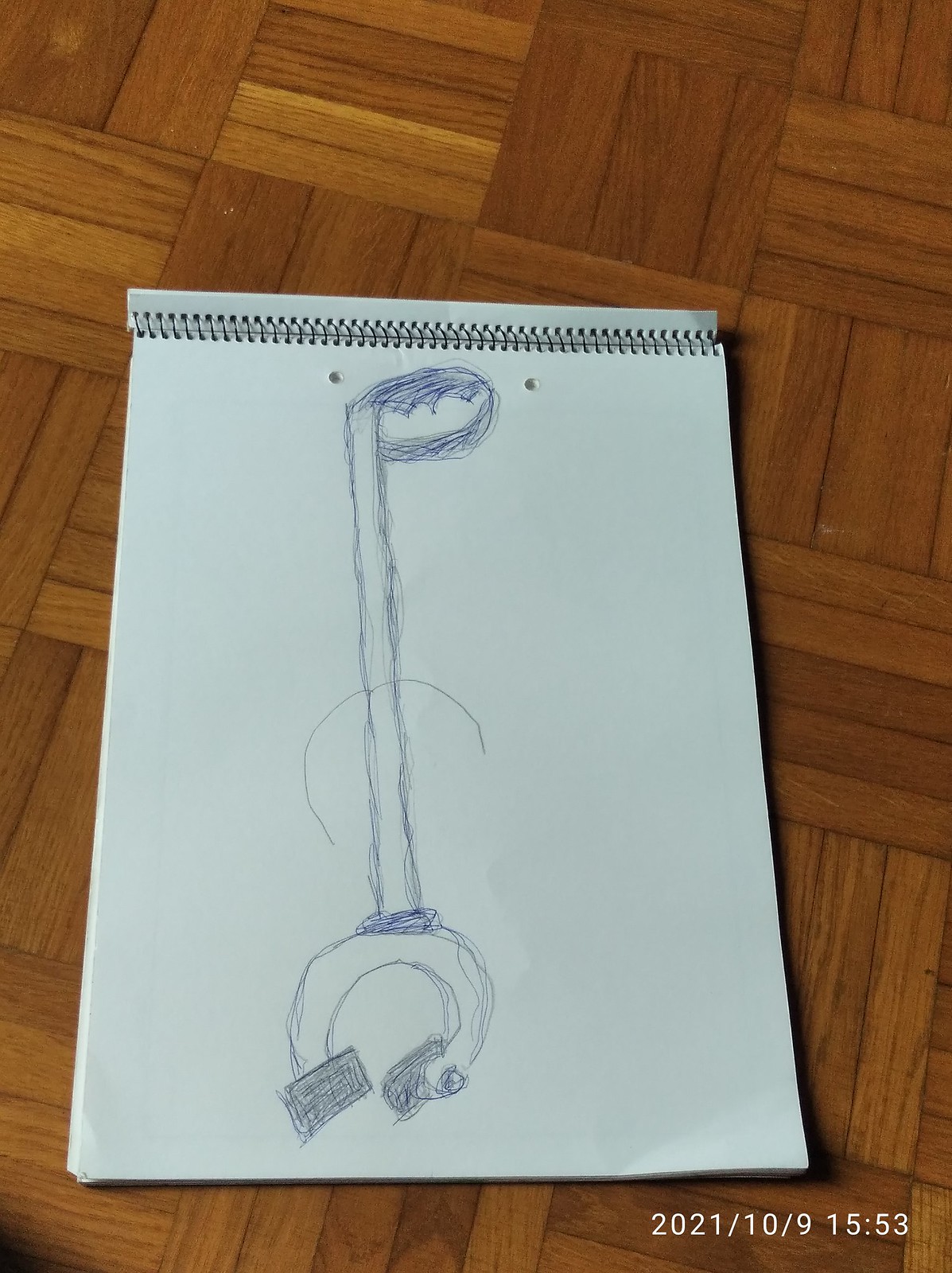A photograph captures an artist's notebook laid out on a wooden parquet tile floor, composed of square-shaped wooden strips. The image is in portrait mode and features a timestamp in white text at the bottom right, reading "2021-10-9 at 15:53." The notebook showcases a detailed pencil drawing of a grabber tool, commonly used for picking up items from the floor without bending over. The sketch meticulously depicts the tool's handle and the two pinchers designed to grasp objects.